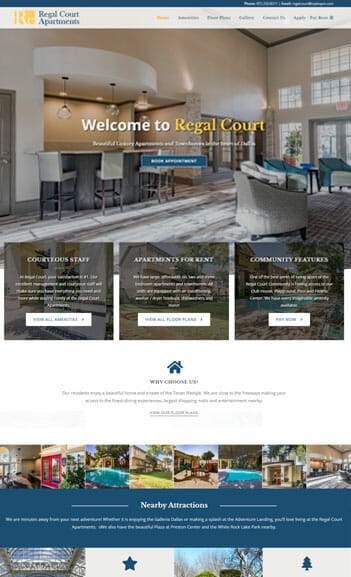The image is a screenshot from a phone showcasing the homepage of Regal Court Apartments. The top of the screen prominently displays "Regal Court Apartments" along with their yellow logo on the left-hand corner. Across the top, there are various hyperlinks which are too small to decipher. Below this, a welcoming message, "Welcome to Regal Court," is overlaid on an image of the apartment lobby. The lobby features a well-decorated space with a luxurious rug, several chairs, and side tables. A bar area with three pendant lights hanging above it adds to the aesthetic appeal of the lobby.

At the bottom section of the image, there are three distinct clickable options labeled: "Courteous Staff," "Apartments for Rent," and "Community Features," each linking to specific pages. Additionally, a collection of images at the very bottom highlights different apartment complexes owned by the Regal Court Company, though the specific apartments are not clearly identified.

Along a blue stripe near the bottom, the text "Nearby Attractions" is written in white, though the detailed text beneath this title is too small to read clearly. The very bottom of the screen also features four icons: an image, a star, another image, and a tree, though these do not appear to be interactive. It seems that the lower portion of the screenshot was cut off, limiting further visibility.